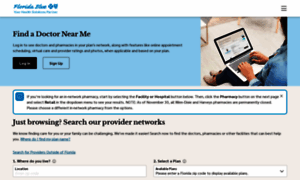This image is a blurry screenshot of a website interface, making most of the text difficult to read. In the top-left corner, there is some blue writing that is illegible. A prominent blue banner across the top displays the text "Find a Doctor Near Me" with some additional unclear writing on the right. Adjacent to this text are the options "Sign In" and "Sign Up." To the right side of the banner, there is a photograph of a woman seated and typing on a laptop resting on her lap. Below this image, there is a long white rectangular box with a blue outline containing unreadable text. Underneath the rectangle, the legible phrase "Just Browsing? Search Our Provider Networks" is visible. Beyond this point, the image's details remain too blurry to decipher. The image is wider than it is tall, and it is devoid of any animals, birds, plants, flowers, trees, mountains, automobiles, motorcycles, bicycles, or helicopters.